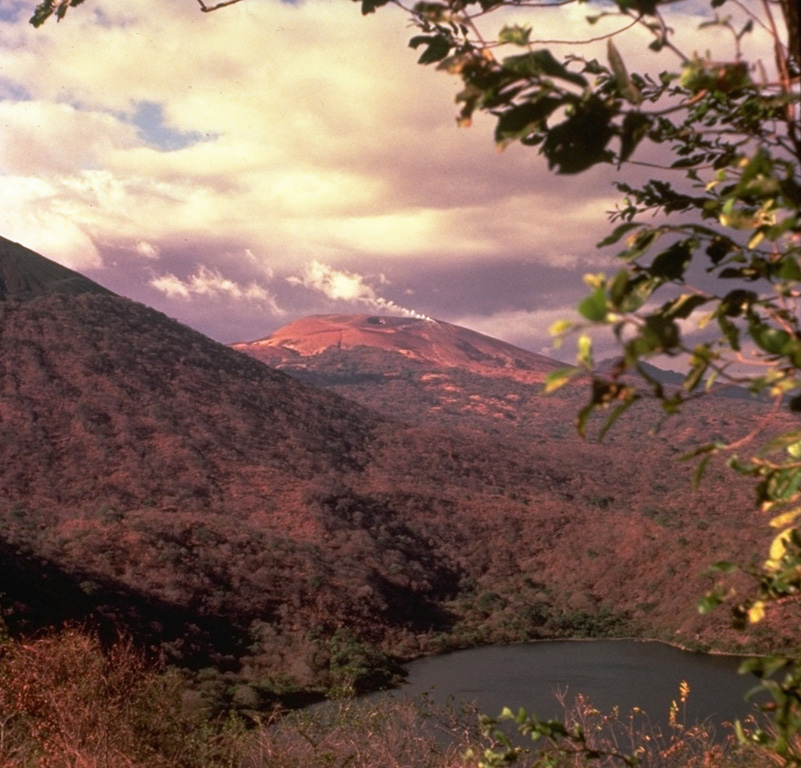A vividly detailed color photograph captures a breathtaking landscape in portrait orientation. The scene features a view across rolling hills toward a distant, steaming volcano or fumarole atop a hill. The reddish-brown pinnacle stands out prominently against the green scrub and forested lower slopes. Suspended overhead, clouds are illuminated by the setting sun, casting a warm, amber glow over the rugged terrain. The perspective is from a hillside vantage point, looking across a valley with an irregularly shaped and dark green body of water positioned at the bottom right. The left side of the image is dominated by a sloping hillside that angles towards the center, flattening into a lush valley below. A large, verdant tree frames the right and top right sections of the photo, adding depth and focus. The foreground is dotted with shrubs, enriching the overall texture and realism of the scene. The meticulous representation encapsulates the serene beauty of nature, with an impressive showcase of vivid trees, undulating hillsides, and the enigmatic steaming volcano devoid of any human or animal presence.